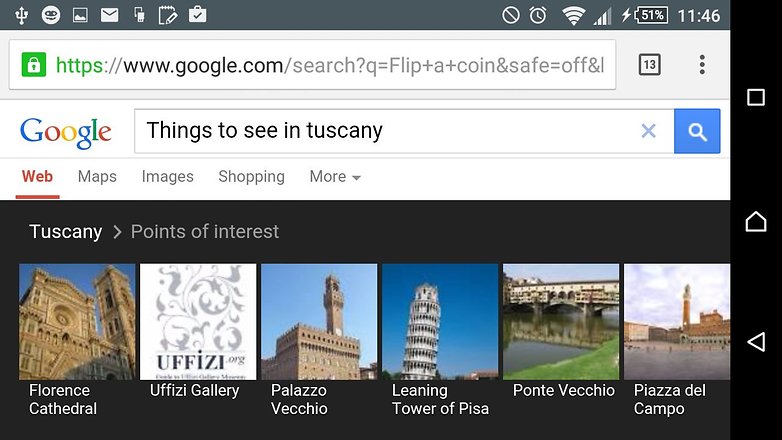This is a detailed screenshot captured from a Google search on a smartphone. The status bar at the top of the screen displays several icons, including a three-arrow icon, a circle icon, a photo icon, an envelope icon, a share icon, a note icon, and a security icon. Additionally, on the right side of the status bar, there are icons for a circle with a line through it, an alarm, signal strength bars, Wi-Fi signal, and battery percentage, which is at 51%. The time displayed is 11:46.

Just below the status bar, there is a search bar with the URL: "https://www.google.com/search?q=FLIP+A+coin&safe=OFFN1." The browser indicates that there are 13 tabs open. This Google search page is focused on "Things to see in Tuscany," with options to navigate through Web, Maps, Images, Shopping, and more tabs.

The search results show various points of interest in Tuscany, each accompanied by a corresponding image. The highlighted points of interest include:

1. Florence Cathedral
2. Uffizi Gallery
3. Palazzo Vecchio
4. Leaning Tower of Pisa
5. Ponte Vecchio
6. Piazza del Campo